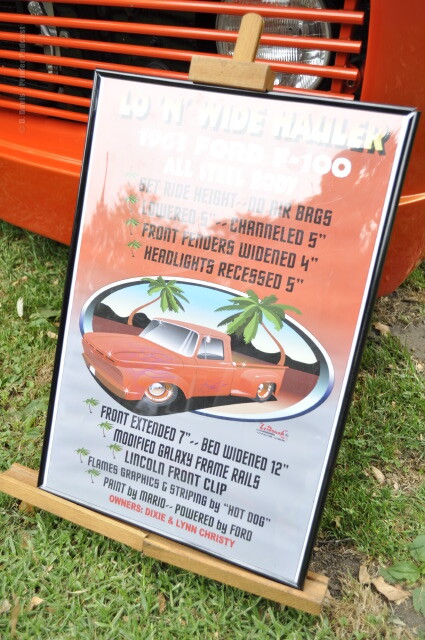The image captures an informational plaque detailing a modified orange 1961 Ford F-100 pickup truck, which is positioned at a car meet or competition, possibly on a grassy area. The focus is primarily on the truck's front right headlight, seen partially due to the zooming. The plaque, leaning against the car, features a cartoonish, almost clip-art-like representation of the truck and is replete with modifications performed on the vehicle. It highlights extensive customizations, such as the bed being widened by 12 inches, the front extended by 7 inches, front fenders widened by 4 inches, and headlights recessed by 5 inches. Notable mechanical and aesthetic enhancements include a modified Galaxy front weight, Galaxy frame rails, a Lincoln front clip, and flame graphics and striping done by an artist known as Hot Dog, with print work by Mario. The truck operates with a Ford engine and belongs to Dixie and Lynn Christie, emphasizing its unique modifications and the craftsmanship involved.